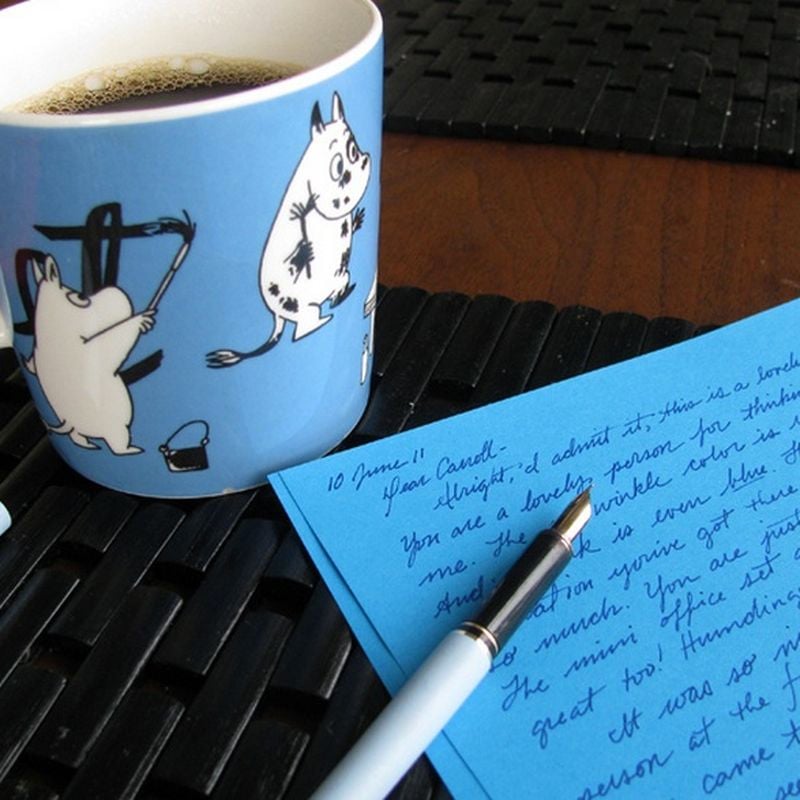The image portrays a serene setup featuring a light blue coffee mug and a handwritten letter, situated on a black placemat atop a brown wooden table. On the left, the light blue mug adorned with illustrations of two white rhinos—one holding a paintbrush and the other covered in paint—is filled to about 80% with dark coffee. To the right, a blue letter written in dark blue ink captures attention, partially visible, with the salutation "Dear Ken Kano" and the date "10 June 11." Resting above the letter is a white pen with a black middle section and a silver tip, adding a touch of elegance to the scene. The black placemat and the wooden tabletop provide a contrasting backdrop that enhances the vividness of the blue elements.